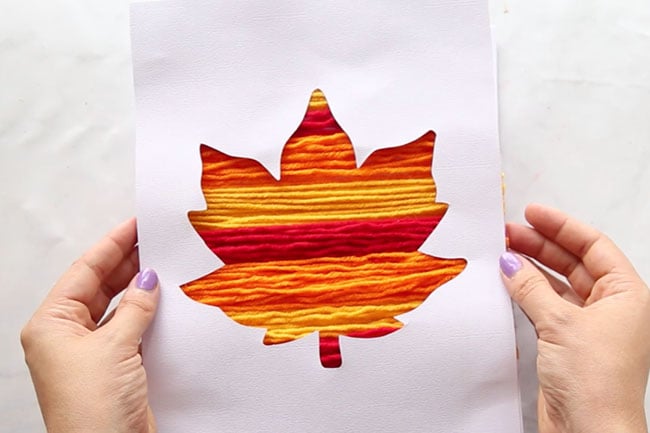In this detailed image, a Caucasian female is holding a white piece of paper with both hands, displaying her purple nail polish. The focal point on the paper is a vividly drawn orange leaf that resembles flames or burning, with hues of orange and yellow. The design features intricate lines that evoke a sense of both fluidity like water and the ethereal quality of clouds. The leaf is prominently sized, with striking and bright details. The background is entirely white, indicating the paper might be placed against a white wall or a tablecloth, emphasizing the colorful artwork on it.